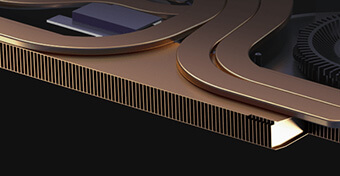This close-up image showcases the intricate cooling system inside a laptop. Dominated by a brass-colored piece extending from the upper left, the scene features a network of thin metal venting tubes designed for ventilation and cooling. These tubes, resembling wavy channels, are arranged vertically and spaced out along the rightward-slanting edge, giving way to a brass-colored surface at the top. Notably, three of these tubes are prominently visible. Starting near the bottom right – just below the center – two tubes arch up and left before curving back toward the top right, while the third one diverges left and exits the frame at the top left.

At the far right of the image, part of a black surface is visible, featuring a round black gear, indicative of the laptop's fan system. Meanwhile, to the left of the brass assembly, there's a dark gray rectangular component with a silver piece underneath. The bottom corners of the image fade into a black background, providing contrast against the metallic components. The center of the image reveals wavy channels that likely serve as part of the laptop's heat sink, enhancing the cooling system's efficiency.